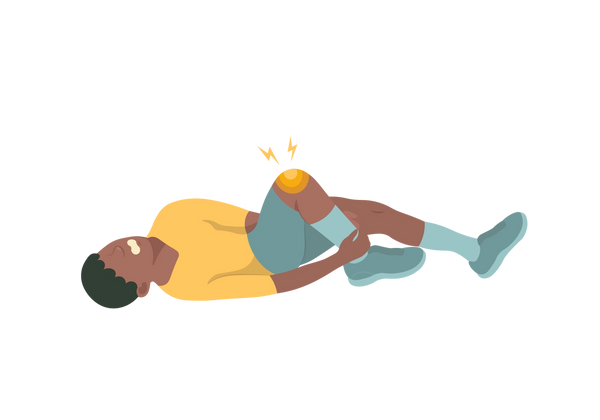The image is a simple, vector-style illustration showing a young boy or man with brown skin, laying on his back against a white background. He has short, curly black hair, and although his eyes are not visible, his mouth is open in a pained expression, possibly gritting his teeth. He is wearing a short-sleeve yellow shirt that reaches his elbows, teal shorts that come just above the knee, light teal socks, and teal sneakers. His left leg is extended outward while his right leg is bent at the knee. The boy is holding his right ankle with both hands. His right knee has yellow and orange concentric half-circles with lightning bolts above it, clearly indicating he is in pain and has injured his knee.